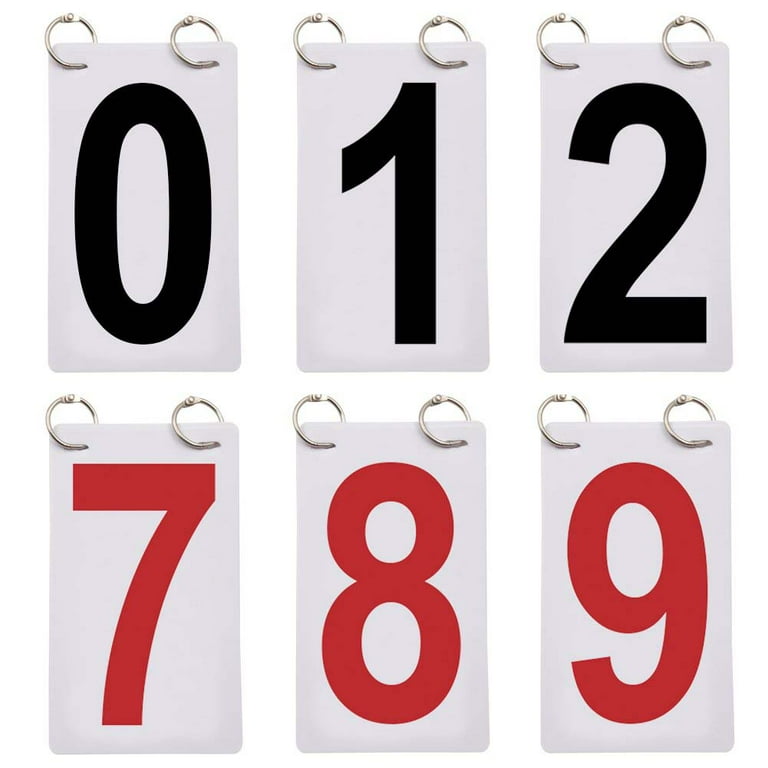The image is square with a white background, displaying a scoring system made up of six vertically rectangular cards, each with numbers on them. These cards are off-white and have two round silver binder rings at the top. The top row of cards, arranged from left to right, features the numbers 0, 1, and 2 in black text. The bottom row, also from left to right, shows the numbers 7, 8, and 9 in red text. The cards appear stacked and capable of folding, with each having a tidy, organized appearance aligned precisely within two vertical columns and three rows.